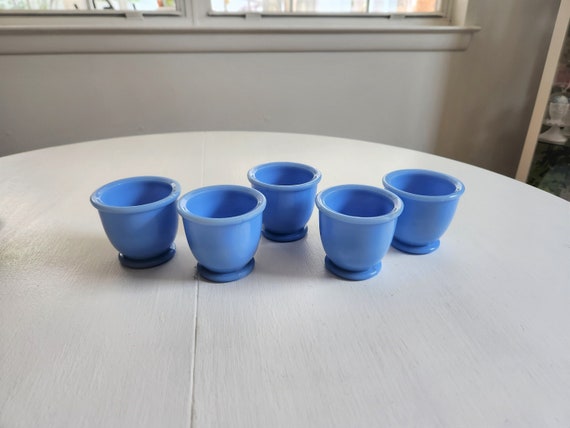The image captures a quaint kitchen scene centered on a circular wooden table, painted white and showing signs of wear. Positioned in front of a partially visible window, the table features five small blue teacups arranged in a pattern reminiscent of the Olympic symbol. Each cup appears to hold approximately four ounces, suitable for a single serving of tea or a shot of ginger. Off to the right side of the photo, slightly cut off, stands a curio cabinet or cupboard, casting a shadow on the wall. This cabinet seemingly holds various items, including a small white figurine. The background wall around the window is a muted gray or khaki color, giving the room a cozy, lived-in feel.